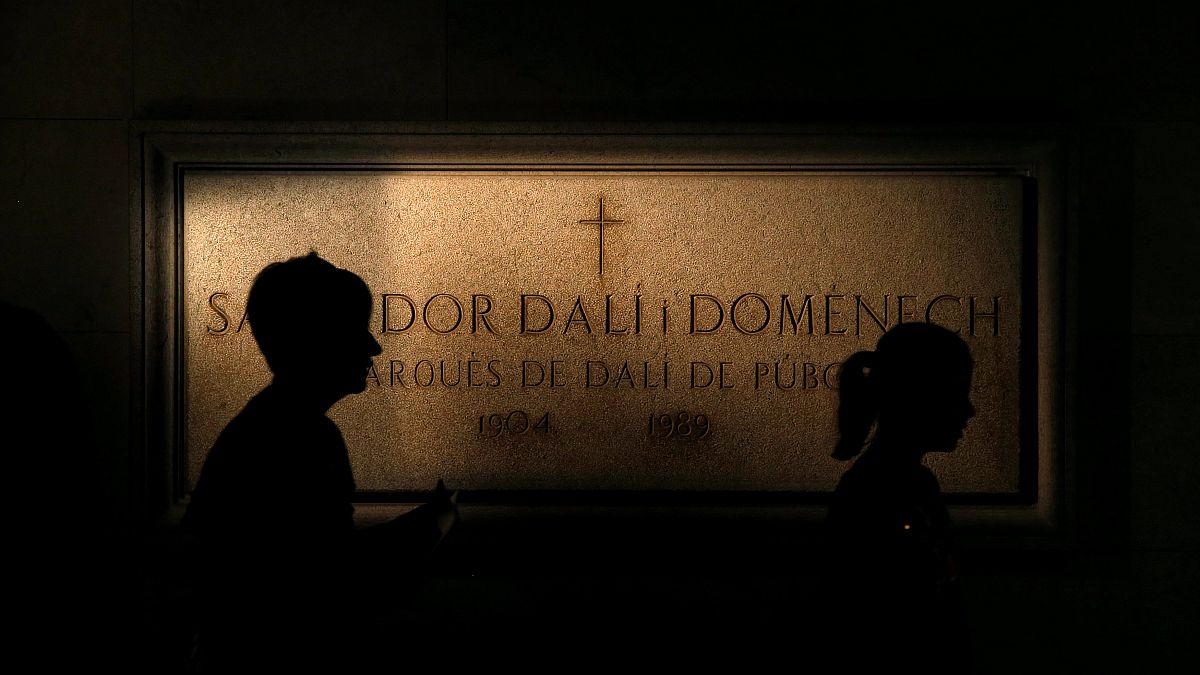The image showcases a gray, metallic-looking window, likely glazed for privacy, reminiscent of those found in bathrooms. This central window features a prominent cross at its core. The main focus is the silhouettes of two people, a man and a woman, walking by the window. The woman, closer to the viewer, has a ponytail, while the man appears further back, possibly holding something. Their silhouettes obscure some of the text on the window, but the visible inscriptions suggest it relates to Salvador Dali, indicating dates from 1904 to 1989, possibly suggesting a memorial or tombstone. The scene is set against a predominantly dark background, with the light source likely coming from behind the window, enhancing the stark contrast of the silhouettes against the light and adding a solemn, shadowed ambiance to the setting.